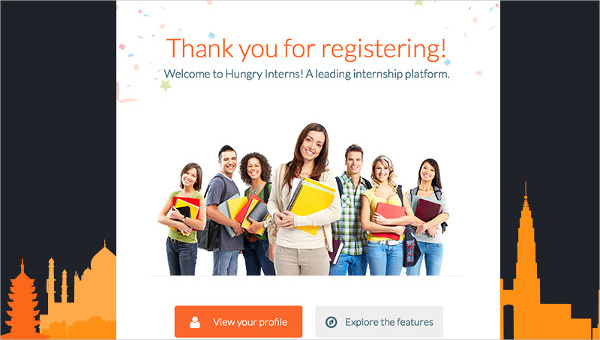The image has a landscape orientation with a posterized silhouette of various iconic city landmarks serving as the backdrop. On the left side of the background, you'll notice structures resembling a pagoda and the Taj Mahal, while the right side features silhouettes of what might be the Empire State Building among other skyscrapers. The background itself is black, contrasting with the shades of orange used for the cityscape silhouettes.

Centrally superimposed onto this cityscape is a nearly square white background. This central element bears the text: "Thank you for registering. Welcome to Hungry Interns, a leading internship platform." Below this welcoming message, a group of young people stand in a line, holding notebooks. Most of them are dressed in blue jeans and are all smiling broadly.

At the bottom of the image, there are two buttons for further interaction. An orange button labeled "View Your Profile" and a white button labeled "Explore the Features."